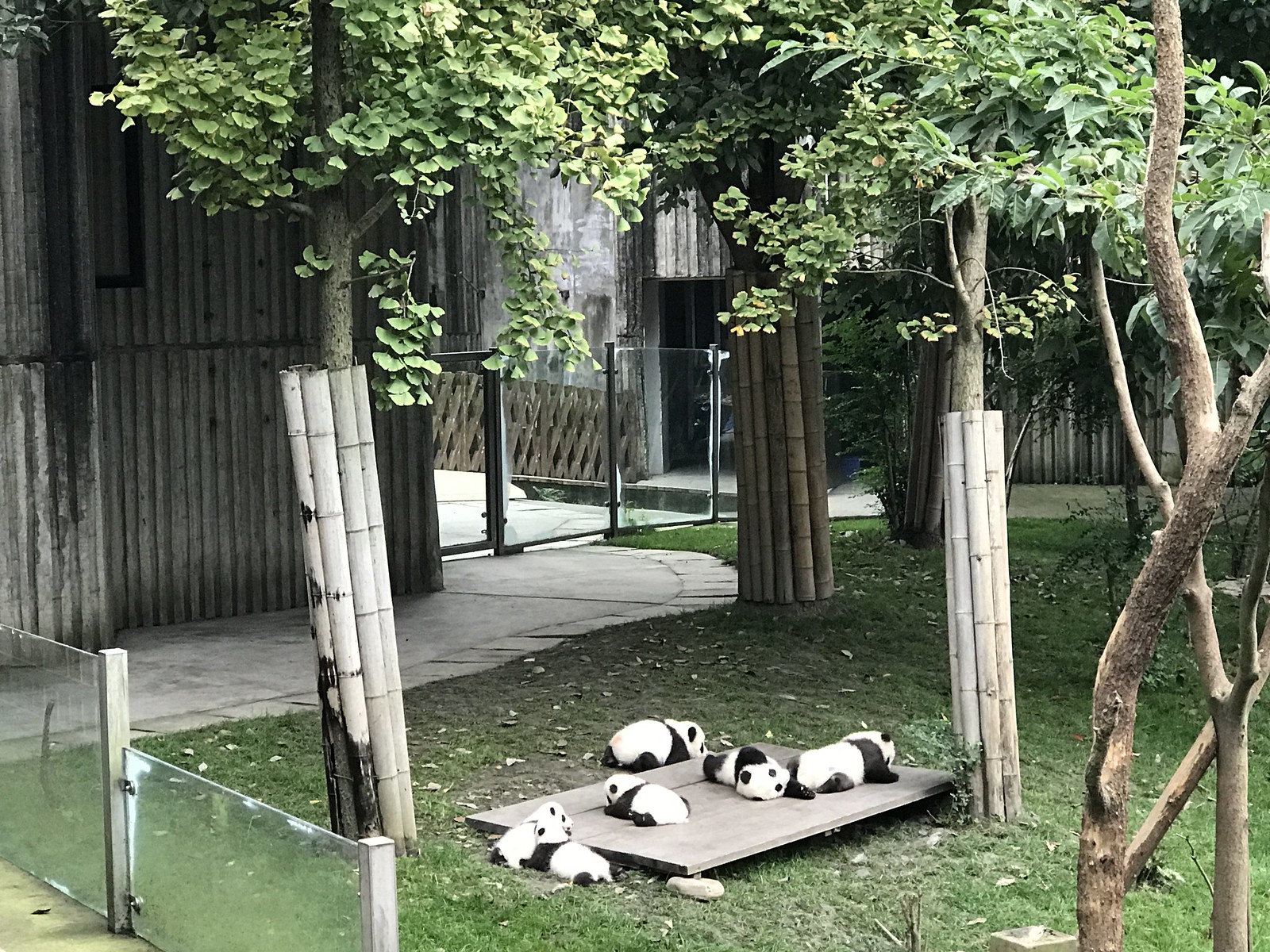This detailed image captures an outdoor panda bear enclosure, likely situated within a zoo or a rescue habitat. The photograph is taken from a vantage point outside and slightly higher than the enclosure itself. The enclosure features a grassy area meticulously maintained with short, green grass. Surrounding the grass are tall trees, each encircled at their bases by bamboo poles — potentially for feeding or tree protection.

In the heart of the enclosure is a raised bamboo wood platform where six or seven young panda bears are gathered. Most of these small, youthful pandas appear to be napping, sprawled comfortably on their bellies, soaking up the sunlight. While a couple of pandas lie close together, touching softly, others are more spread out on the platform. One panda lounges near the platform's edge, with just its fur gracing the bamboo wood.

The entire enclosure is secured by a glass fence, ensuring the pandas' safety and visibility for visitors. Additionally, a concrete walkway traces along the perimeter, lined with more trees and bamboo. In the background, the scene broadens to reveal additional glass fencing, some wood fencing, and adjacent buildings, possibly used for panda care or logistical support. This serene snapshot highlights both the pandas' natural behaviors and the thoughtfully designed habitat created for their well-being.